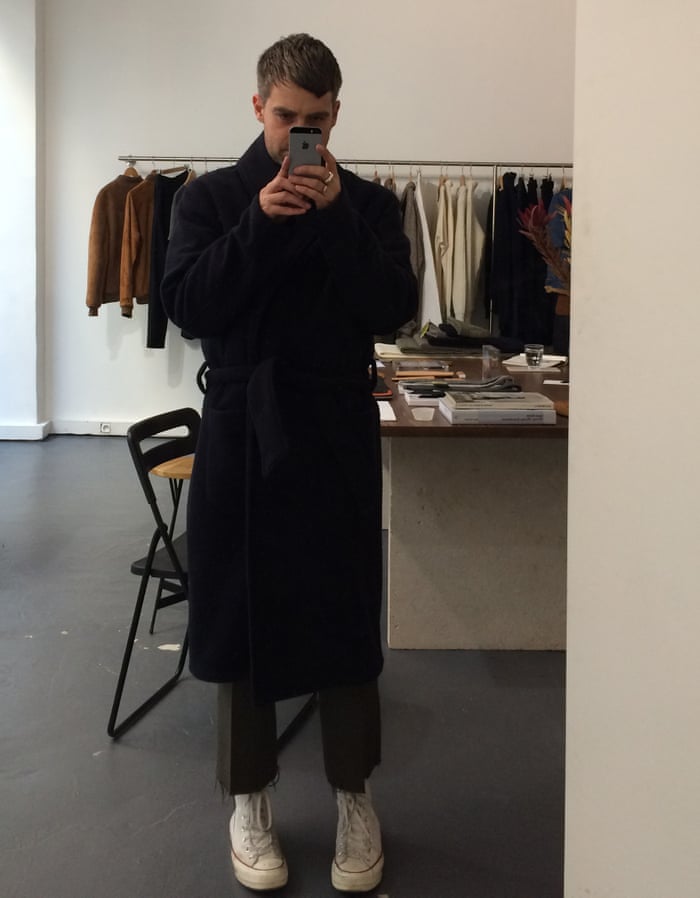In this color portrait-oriented selfie, a man around 30 years old stands in front of a mirror, capturing his outfit with a cell phone camera held near his face. He has short, dark brown sideswept hair and is wearing a long, dark trench coat that extends to his knees, paired with dark grey pants and slightly dirty white high-top sneakers, featuring a platform base. The background reveals a white wall and a dark grey or black concrete floor. To the man's right, there is a row of garments, including brown jackets and white shirts, hanging on a coat rack. To his left behind him sits a neatly organized desk with various books and papers stacked on top, accompanied by a black metal chair, suggesting an office or retail environment. The overall photographic style is realism.